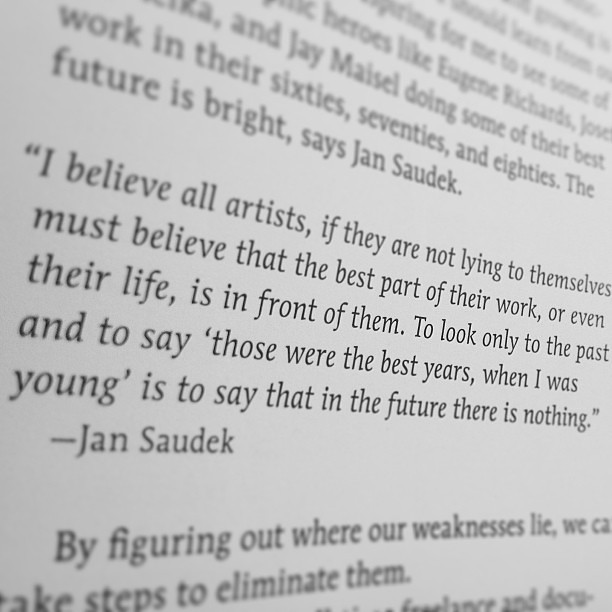On a light gray background, this black-and-white print piece features printed text at the top that becomes blurrier as it ascends. The first clearly legible line reads, "...Ann J. Maisel doing some of their best work in their 60s, 70s, and 80s period. 'The future is bright,' says Jan Sadek." Below this, a fully readable paragraph in quotation marks states, "I believe all artists, if they are not lying to themselves, must believe that the best part of their work, or even their life, is in front of them. To look only to the past and to say those were the best years when I was young is to say that in the future there is nothing." This quote is attributed to Jan Sadek. Following this, another visible line says, "By figuring out where our weaknesses lie, we see a..." though the rest is cut off. Below that, it appears to state, "take steps to eliminate them."